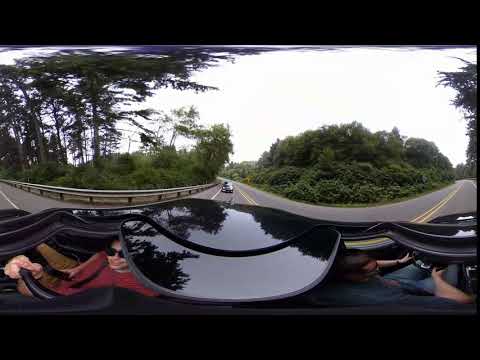This is a fisheye-distorted, panoramic image capturing the interior of a car in motion on a black asphalt road. The photograph appears flattened, commonly seen in 360-degree images. The image features two people: The driver on the right, with short dark hair, wearing a dark blue shirt and jeans, with both hands on the steering wheel. The front seat passenger on the left is wearing sunglasses, a red shirt, and tan pants while holding a black selfie stick protruding through the sunroof. Behind their car, another vehicle is visible. The road they are traveling on has yellow median lines and white shoulder markings, indicating it is a two-lane road. On the left side, a silver guardrail borders the pavement, backed by tall green trees and bushes. The right side is lined with a similar dense green foliage but of shorter trees. The sky above appears white and overcast, creating a bright but hazy atmosphere.